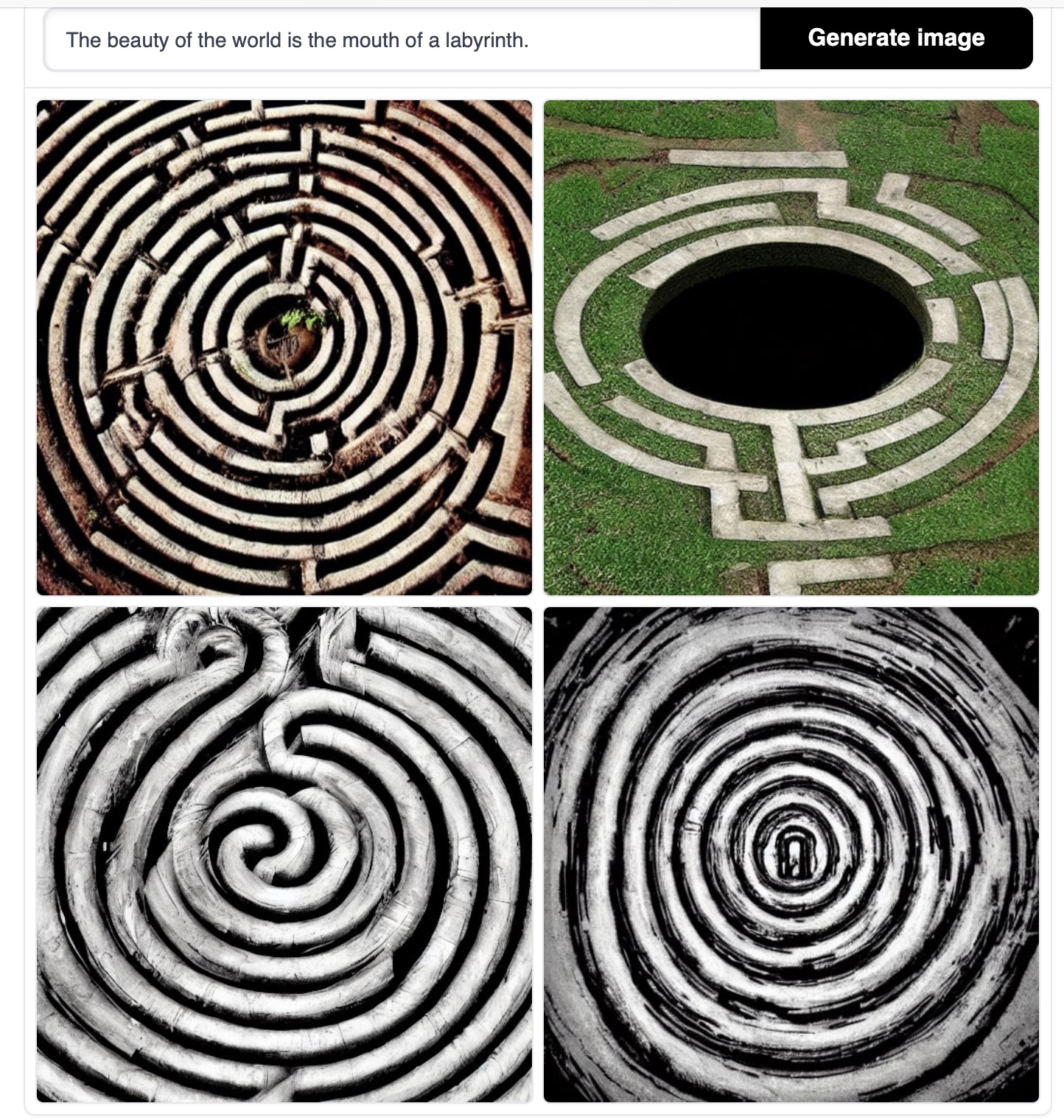This image is a top-down compilation of four distinct maze illustrations, displayed in a search engine interface with the text "the beauty of the world is a mouth of a labyrinth" in the search bar and a "generate image" button above. In the upper left quadrant, there is a black-and-white aerial view of a circular labyrinth, layered meticulously with walls and featuring some greenery at the center. The upper right corner shows a flat, glyph-like labyrinth set within a grassy area with a prominent black center, bordered by white stones. The bottom left image portrays a labyrinth constructed from plant roots, coiled intricately to resemble a maze, while the bottom right showcases a silver and black labyrinth resembling a spiral or tornado shape. The entire composition reflects a variety of labyrinth designs, emphasizing the intricate beauty and complexity inherent in each depiction.